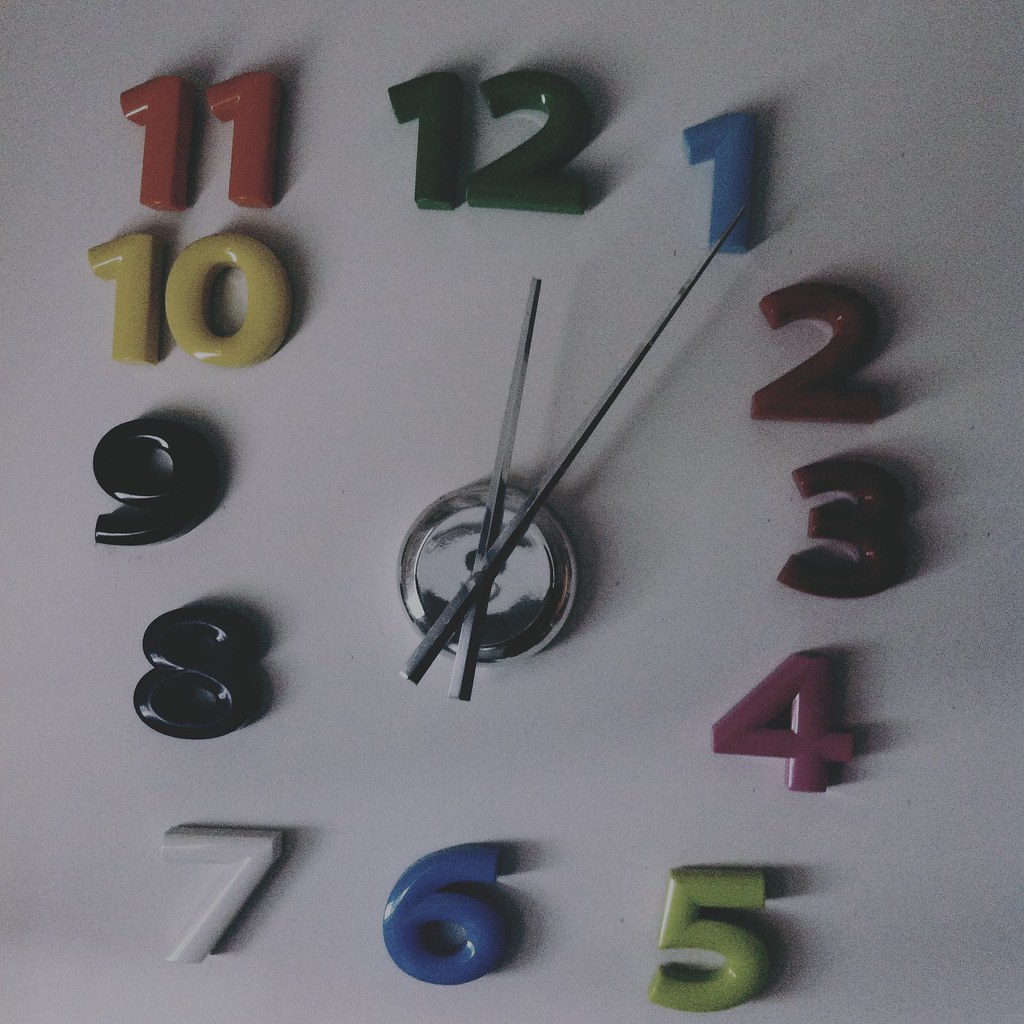This image showcases a creatively designed clock affixed directly to a white living room wall, appearing almost as if it were pasted on. The clock lacks a traditional border or outline, with its defining feature being a central chrome circle from which emanate sharp, stainless steel hour and minute hands. The hour hand points just to the right of the 12, and the minute hand is just past the 1, indicating the time is approximately 12:06. The numbers marking the hours are formed by colorful plastic blocks, much like those found in a kindergarten setting. Each number is distinct in color: the 12 is dark green, the 1 is light blue, the 2 is dark red, the 3 is another shade of red, the 4 is pink, the 5 is light green, the 6 is dark blue, the 7 is white, and both the 8 and 9 are black. The 10 is yellow, and the 11 is orange. Each number is arranged in a circle and casts subtle shadows on the wall, giving depth to the design. The ambient lighting in the room casts a slight shadow, skewing the overall hue of the wall to a grayish tone.